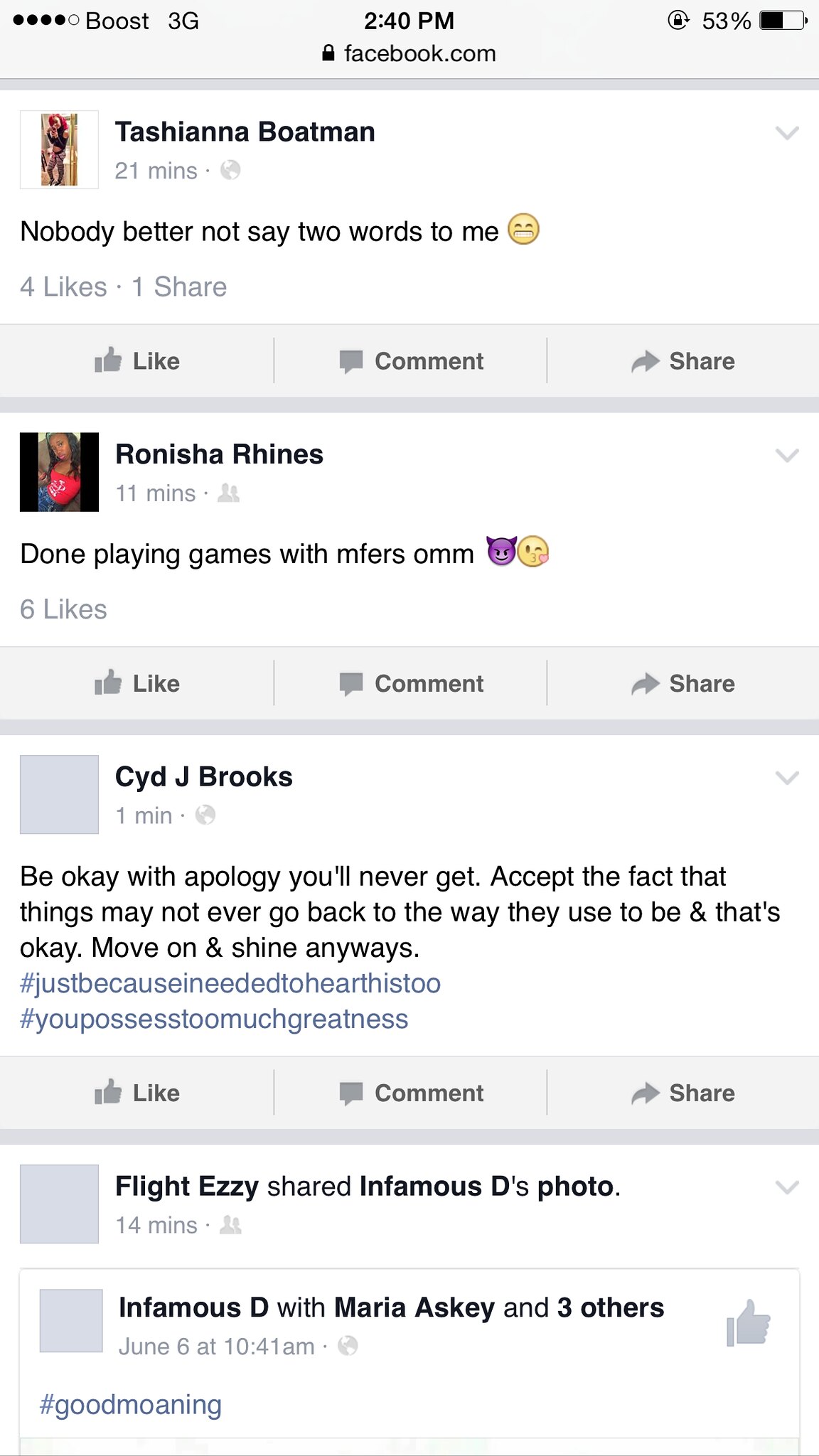The image is a color screenshot of the Facebook mobile app displayed in portrait orientation, captured at 2:40 PM with a battery life of 53%. At the top of the screen, "Facebook.com" is prominently featured in black type against a gray horizontal band. Below it, there are three distinct posts. The first is from Tashiana Boatman, timestamped 21 minutes ago, stating emphatically, "Nobody better not say two words to me," accompanied by a straight-faced emoji. The second post, from Ronisha Rhines, features text saying, "Done playing games with MFers, OMM," and includes both a devil sign and kissy face emoji, with six likes received. The third post is a longer motivational message from Sid J Brooks, encouraging acceptance and personal growth: "Be okay with apology you'll never get, accept the fact that things may not ever go back to the way they used to be and that’s okay. Move on and shine always," followed by hashtags #justbecauseIneededtohearthis and #youpossesssomuchgreatness. Additionally, there is a notification at the bottom stating, "Flight Easy shared Infamous D's photo," involving Maria Esky and three others. Underneath each post are the standard "like," "comment," and "share" buttons with gray icons.